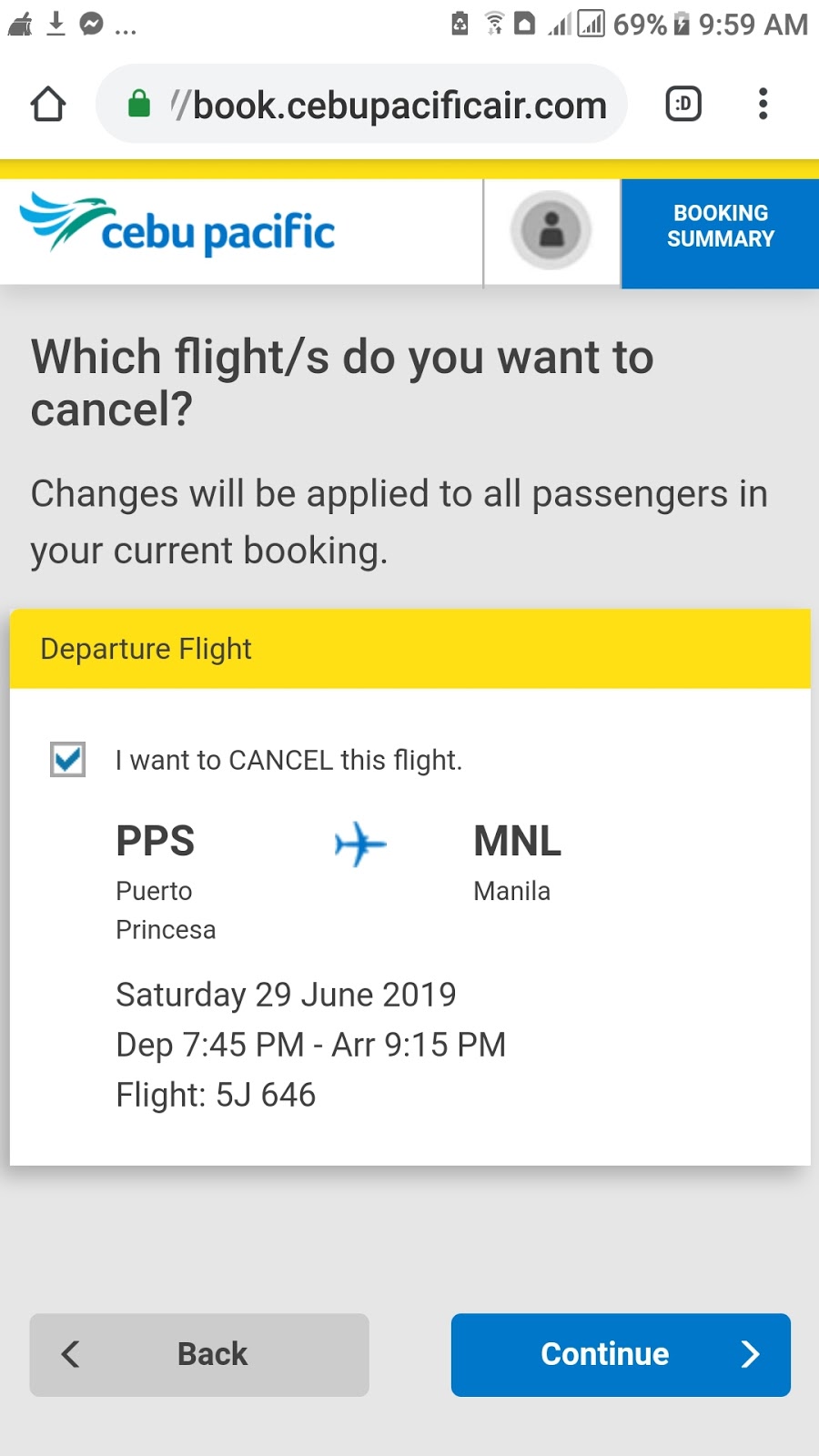In this screenshot, the upper right corner displays standard mobile interface icons, including battery life, Wi-Fi signal, cellular reception, and the time at 9:59 a.m. Directly below is the browser's address bar showing the URL "book.cebupacificair.com" highlighted with a yellow underline.

Dominating the top third of the image, there's a banner featuring the Cebu Pacific logo in blue and green, accompanied by the text "Cebu Pacific" in bold blue font. Adjacent to this, within a blue square in the upper right corner, the text "Booking Summary" is prominently shown.

Underneath, set against a gray background, black text asks, "Which flight do you want to cancel? Changes will be applied to all passengers in your current booking." A yellow banner indicating “Departure Flight” separates the sections.

Below this yellow banner, there is a white box detailing the flight information: 
- The statement "I want to cancel this flight: Porto Princesa to Manila."
- An icon of a blue airplane is placed between the two locations.
- The flight details specify it is scheduled for Saturday, 29th June 2019, with a departure time of 7:45 p.m. and an arrival time of 9:15 p.m.